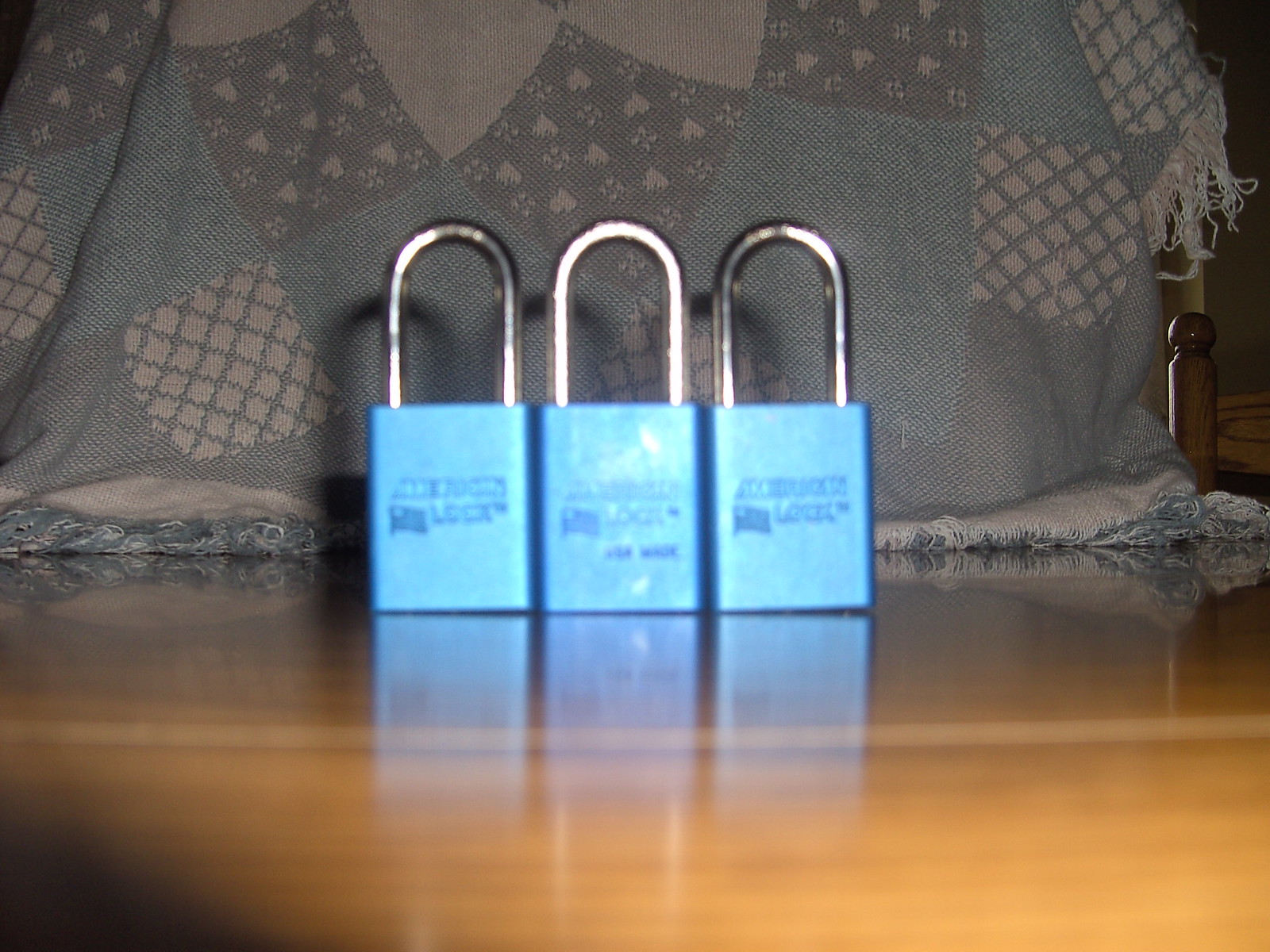The image depicts three blue padlocks standing upright in a row on a wooden table or countertop. Each padlock has a tall, stainless steel, U-shaped shackle, gleaming under the light, indicating they are in a locked position. Engraved on the front of each padlock is the word "LOCK" along with "USA made" and an indistinct flag symbol as part of the logo. Behind the padlocks, a draped blanket is visible, featuring a patchwork design with criss-cross patterns and heart shapes. The blanket's colors are muted, including light pink or beige, light blue, and very light brown. The scene is slightly blurry, adding a subtle softness to the overall composition.